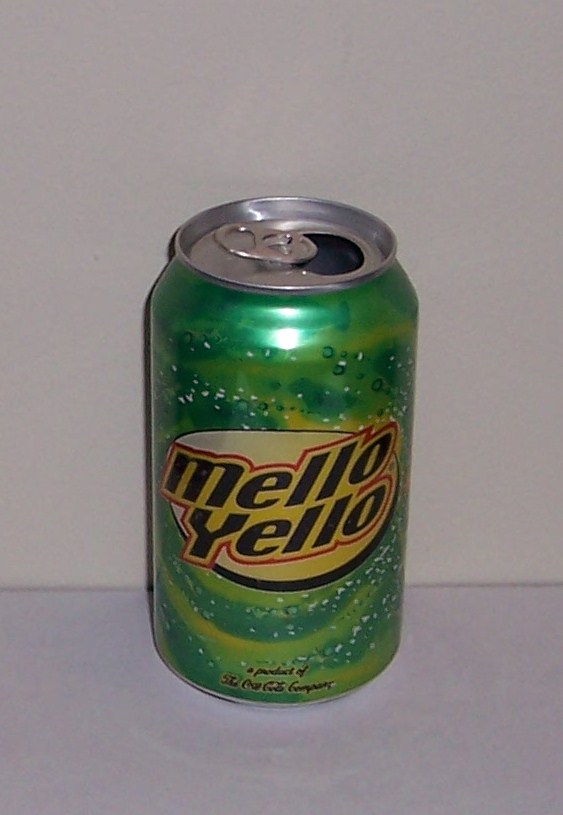This is a color photograph of an opened Mellow Yellow soda can sitting on a white table against a white wall. The can features a design with light and dark green swirls and yellow streaks. The logo, prominently centered, consists of the words "Mellow Yellow" in black letters outlined in red, displayed over a yellow circle. Below, in black text, it reads "A product of The Coca-Cola Company." The image also captures the reflection of the camera's flash on the top middle part of the green section of the can. The tab is pulled back, indicating that the can has been opened, and it appears to have been partially consumed.